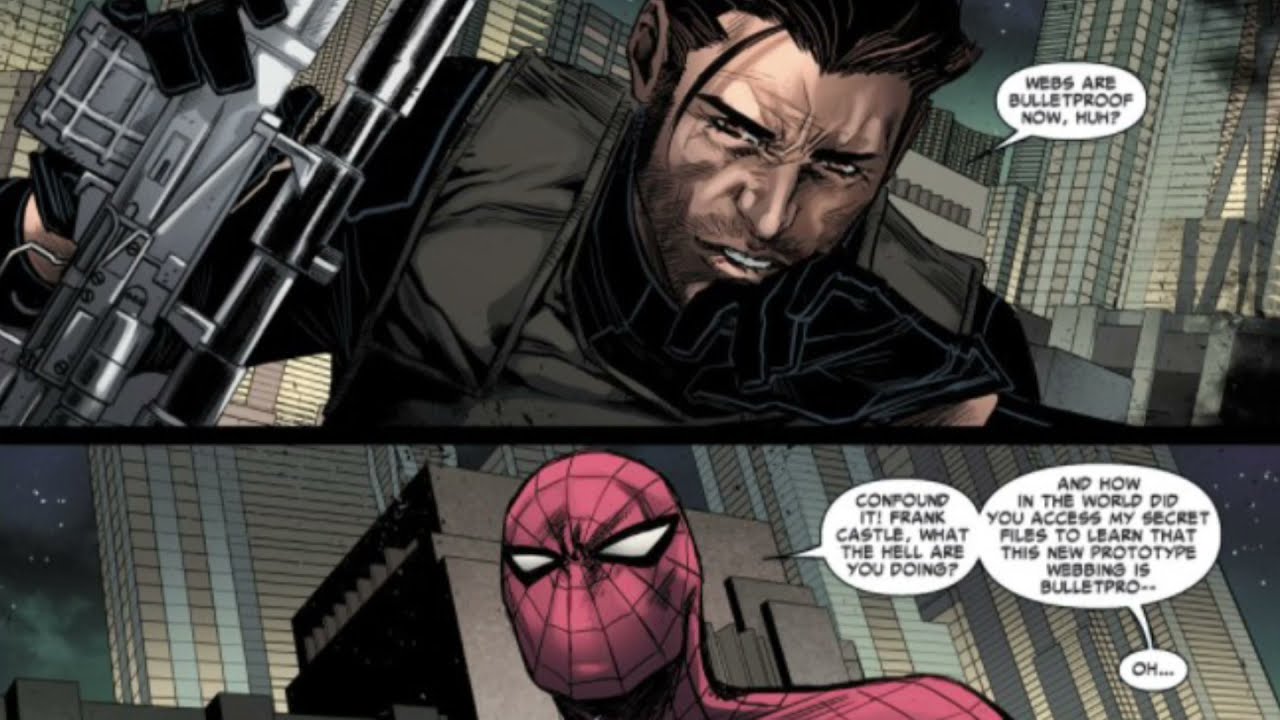The image is a detailed panel from a Spider-Man comic, divided into two distinct sections—the upper panel is significantly larger than the bottom one. In the top portion, a stern-looking man wearing black armor-like clothing and a black glove on his left hand is depicted. He has short black hair, a five o’clock shadow, and dark, scrunched eyebrows that emphasize his fierce demeanor. His left hand touches his bottom lip, partially exposing his upper teeth, while his right hand grips the trigger part of a rifle equipped with a scope. The man, identified as Frank Castle, stands against a backdrop of high-rise buildings in various shades of gray. A speech bubble from him reads, "Webs are bulletproof now, huh?"

In the bottom, smaller section, Spider-Man is shown from the shoulders up, facing the viewer in his classic red costume with white eyes outlined in black. His background also features grayish high-rise buildings at different heights, and the night sky is marked by scattered white stars. Spider-Man's word bubble states, "Confound it, Frank Castle! What the hell are you doing? And how in the world did you access my secret files to learn that this new prototype webbing is bulletproof, oh!" This detailed panel captures the intense confrontation between Spider-Man and Frank Castle, set against a nighttime urban backdrop.